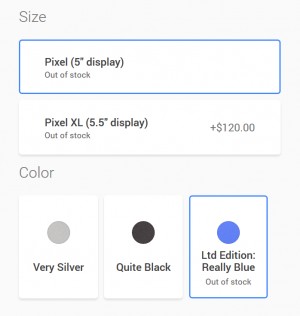This image is a screenshot of a menu interface designed for selecting options while purchasing a Google Pixel smartphone. The interface is set against a light gray background with text in a slightly darker gray font. At the top, it prompts the user to choose a "Size" for the phone. 

The first option presented is within a white box with a blue border, reading "Pixel 5-inch display - Out of Stock." Directly below it is another white box, indicating "Pixel XL 5.5-inch display - Out of Stock" with an additional note specifying a price increase of $120 for this model.

Further down, the menu provides color options, indicated by the word "Color" in gray font. The choices available are "Very Silver," "Quite Black," and "Really Blue." The "Really Blue" option, noted as a limited edition, is marked "Out of Stock" and is also highlighted by a blue border, indicating it might have been selected previously.